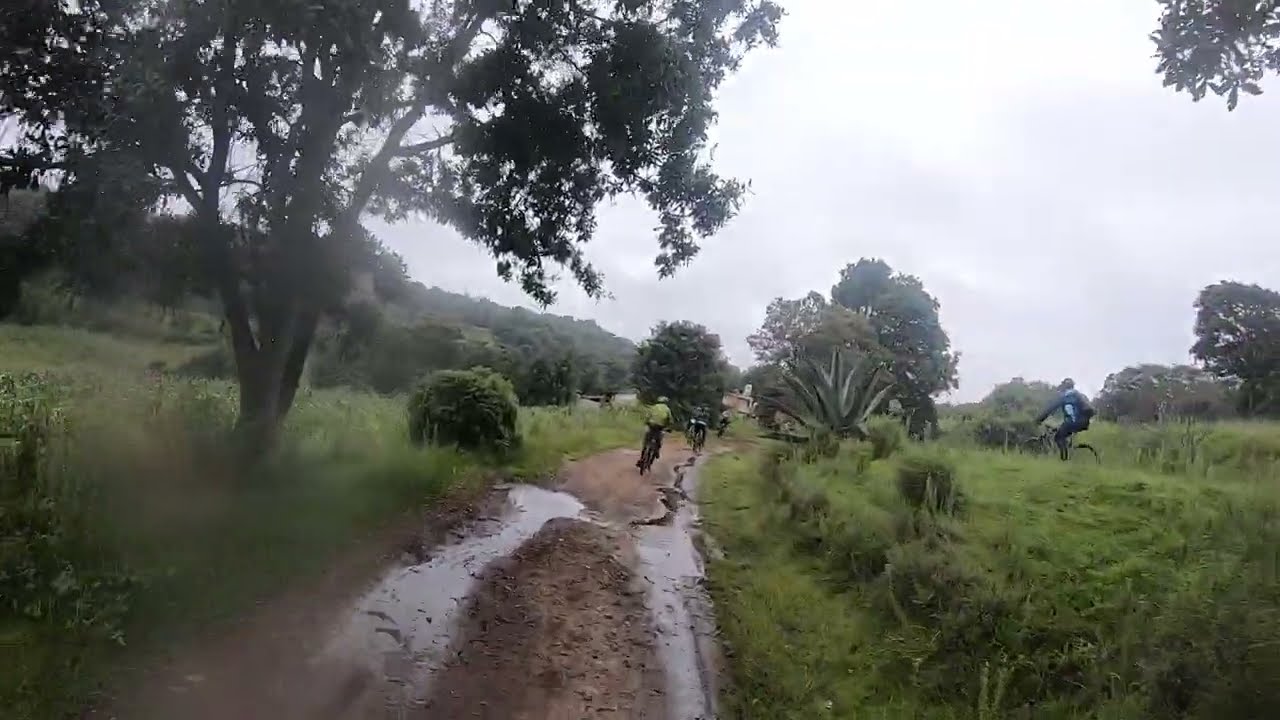The image captures a muddy dirt path cutting through the center, bordered by tall, overgrown green grass and varied vegetation. The road is filled with dark grey puddles, completely soaked from the recent rain. On either side, the lush greenery is mixed with bushes and a big tree on the left, creating a somewhat hilly landscape. The sky overhead is a dark grey, heavy with clouds, rendering the scene overcast and hazy. In the middle of the road, three cyclists can be seen clearly; the closest to the camera is in a yellow jacket, while the other two further back are in grey or white, all riding black bicycles. On the right side, riding through the grass, another cyclist wears a blue and white outfit, also on a black bike. The background and edges of the image are filled with more tall grass and sporadic bushes, completing this dynamic, nature-immersed scene.